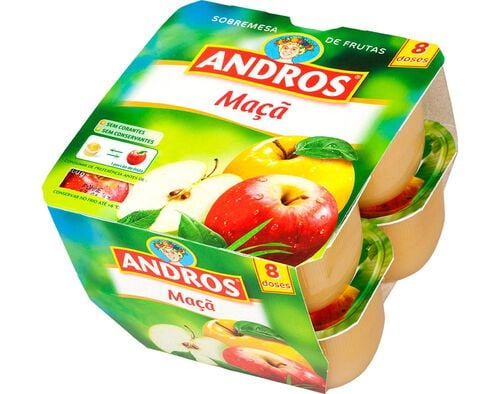The image depicts pre-packaged applesauce under the brand name "Andros". The brand is prominently displayed within a red flag that is outlined with a yellow border. The Andros logo features a person with pale skin adorned with a crown made of various colorful fruits. The packaging is predominantly green and showcases an appealing assortment of apples in the lower right corner: a vibrant red apple in the foreground, a yellow apple with a green leaf partially visible behind it, and a sliced apple with white flesh beside the red apple. The label includes the word "maca," which, based on context, appears to be the term for apple in the language used on the packaging. Indicators on the top right reveal that the package contains eight individual containers. The applesauce, visible through the transparent sections of the containers, appears to be a beige color, suggesting a traditional applesauce texture.